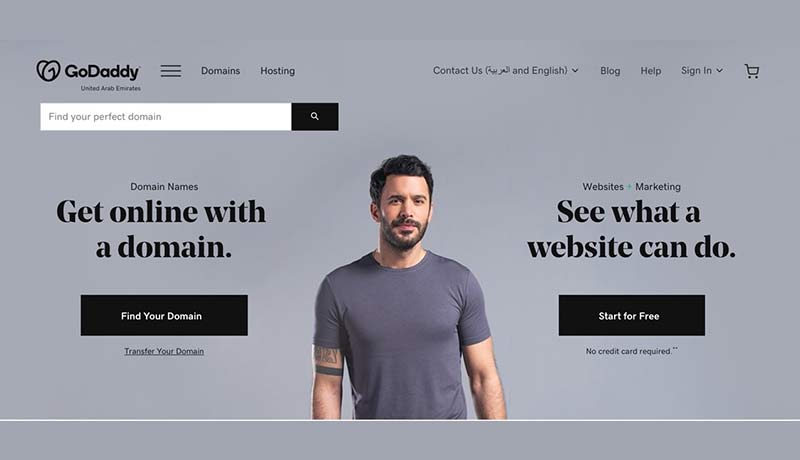This is a detailed landscape-oriented photo of the GoDaddy website's home page, set against a gray background. The main frame is bordered at the top and bottom by thin white lines, creating a rectangular shape with gray margins.

At the top of the home page, within a white border, is the GoDaddy logo, which combines a stylized "G" and "D". Next to the logo, it reads "United Arab Emirates," followed by a hamburger menu on the right-hand side. Additional navigation options include "Domains" and "Hosting." A "Contact Us" link is displayed in Arabic and English, alongside a language selection dropdown indication.

Further to the right, the top navigation bar includes links labeled "Blog," "Help," and "Sign In," each with a dropdown caret for additional options, plus a shopping cart icon.

Beneath this header is a prominent, white rectangular search box accompanied by a black magnifying glass icon. The placeholder text within the search box reads, "Find your perfect domain." 

Below the search bar, the section "Domain Names" features promotional text: "Get online with a domain" and includes a black button with white text, "Find your domain." An image of a man with a beard and tattoo on his right arm, dressed in a gray shirt, appears below the text.

To the right of this image, the section titled "Websites Marketing" prompts users with, "See what a website could do," and offers a black button with the text, "Start for free, no credit card required."

This home page snapshot effectively showcases the main features and services offered by GoDaddy, packaged in a clean, intuitive layout.